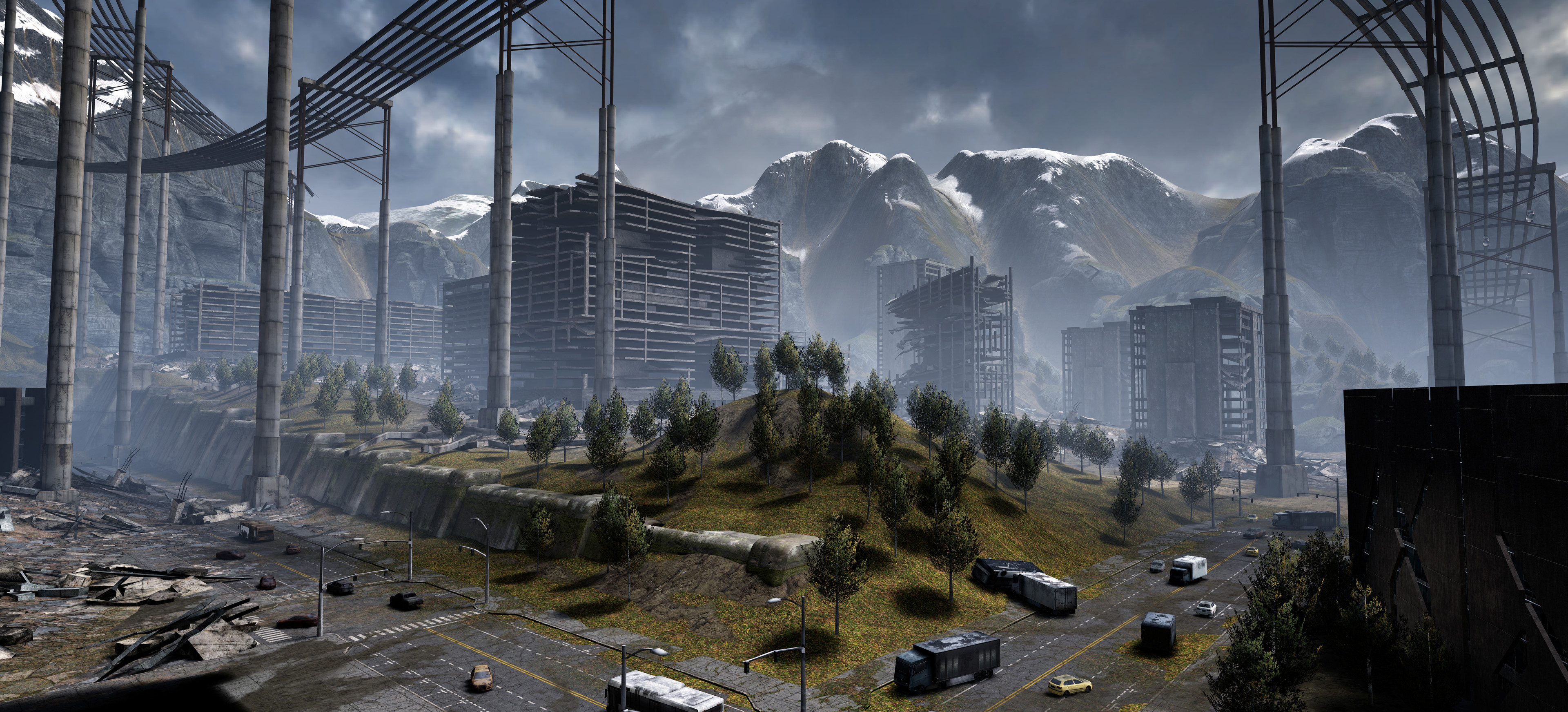The image depicts an apocalyptic cityscape ravaged by disaster. In the foreground, there are overturned vehicles, including cars and buses, scattered haphazardly across a damaged roadway. Toward the left, debris is strewn about from what appears to be a destroyed structure, amidst gray pillars supporting multi-directional tracks, hinting at the remains of a bridge. The middle ground reveals high-rise buildings heavily damaged, with blown-out windows and walls, enveloped in thick, rolling smoke and dark gray clouds. A subdued greenery adds a touch of life, yet it appears unhealthy and bleak. In the distance, the snow-capped mountain range stands tall under an overcast and ominously dark sky, despite it being the middle of the day. The overall scene has a surreal, computer-generated feel, evoking a sense of simulated catastrophe rather than a real photograph.